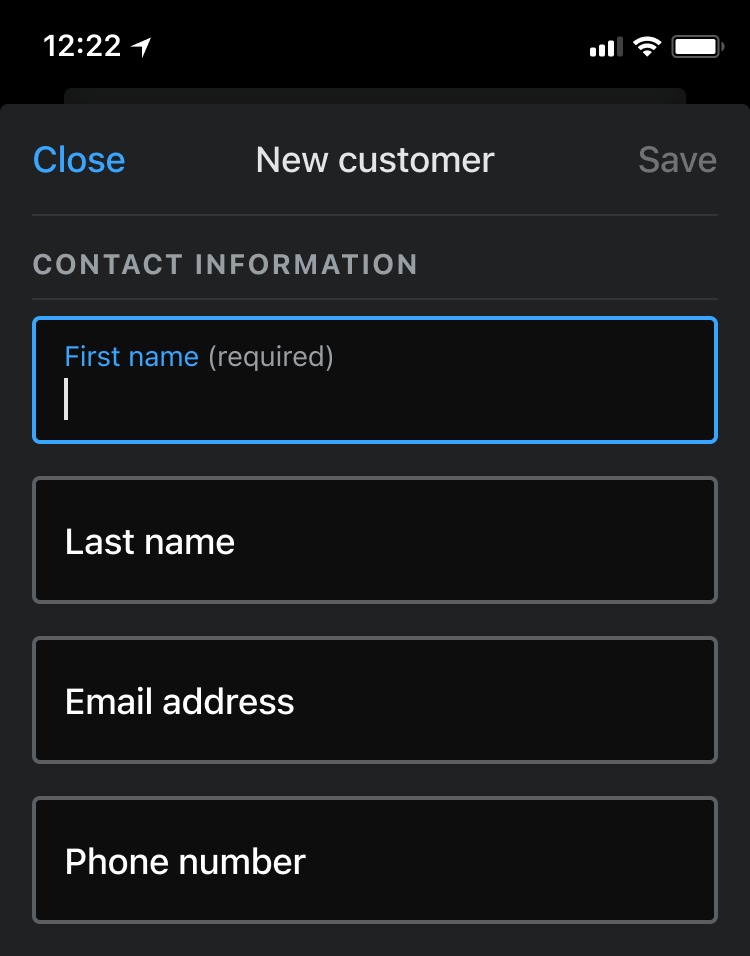The screenshot displays a user interface from an iPhone with a predominantly black background. At the center of the screen, there is a blue button labeled "New Customer." Above this button, in gray text with outlined capitals, reads "Save Customer Information." Below this section, the interface prompts the user to input the "First Name," indicated as a required field in parentheses, where the cursor is currently positioned.

Following the first name input field, there are additional fields for "Last Name," "Email Address," and "Phone Number," all outlined in gray with white text on the black background. 

In the status bar at the top of the screen, on the left side, the time is 12:22 PM, and next to it is the location services icon, indicating that location services are active. On the right side of the status bar, the signal strength shows three out of four possible bars, the Wi-Fi icon indicates that Wi-Fi is enabled, and the battery is fully charged at 100%.